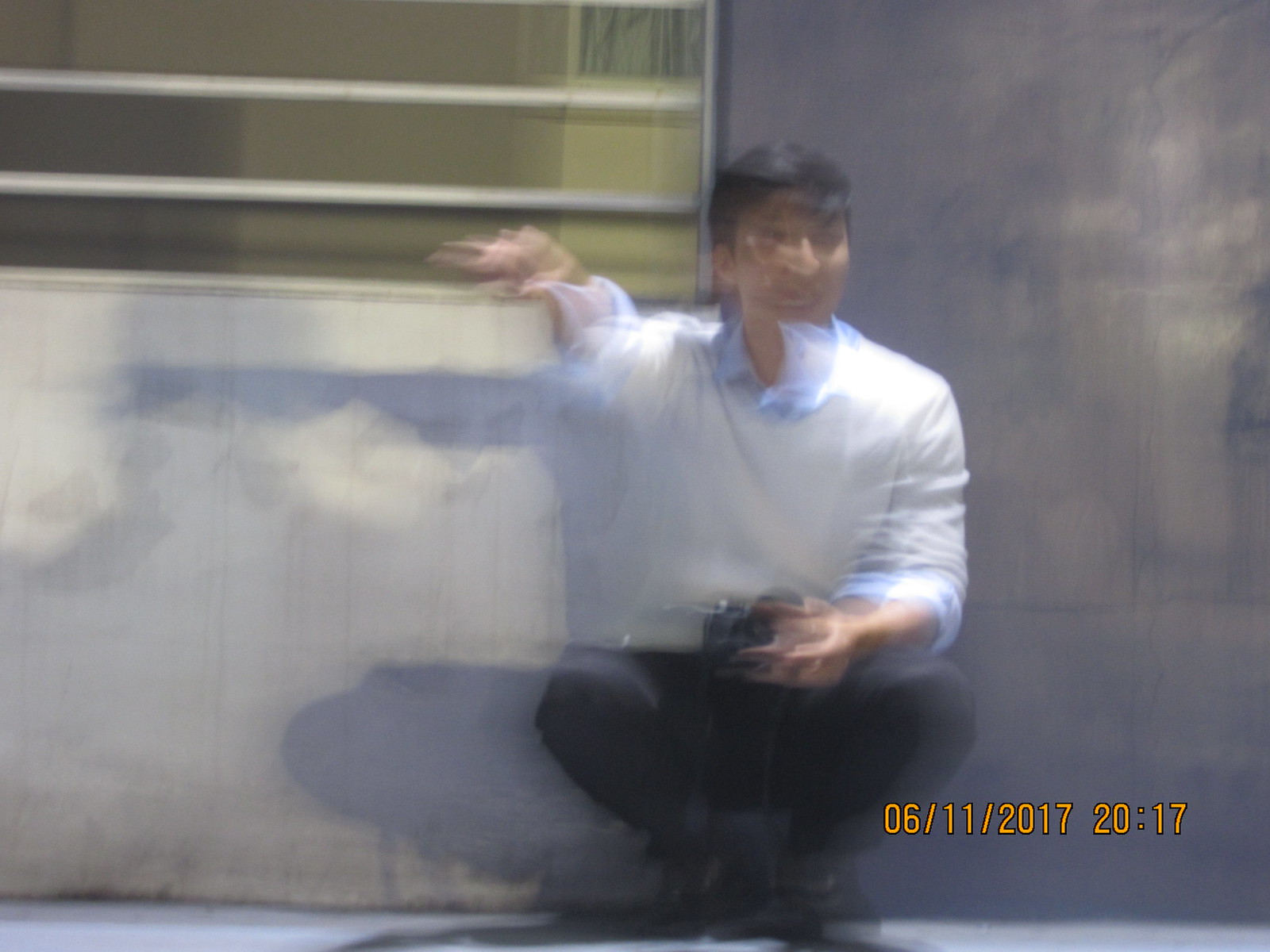A blurred photograph shows an Asian man with short, straight black hair, squatting on the ground. He wears black pants and a light blue long-sleeve dress shirt with slightly rolled-up sleeves, layered under a cream-colored, V-neck sweater. His dark sneakers are visible, and he appears to be holding a black object in his left hand, possibly a camera or a smartphone, near his midsection. His right hand is resting on top of a cement wall, which has two horizontal gray bars above it. The man is facing the camera but is slightly turned to the right. Behind him is a dark gray wall that extends upward, and above his left shoulder are light gray horizontal window frames with thin white banisters. The image is illuminated from above, further washing out details, and there is a yellow timestamp at the bottom of the photo that reads "06/11/2017 20:17," indicating it was taken on June 11, 2017, at 8:17 PM.